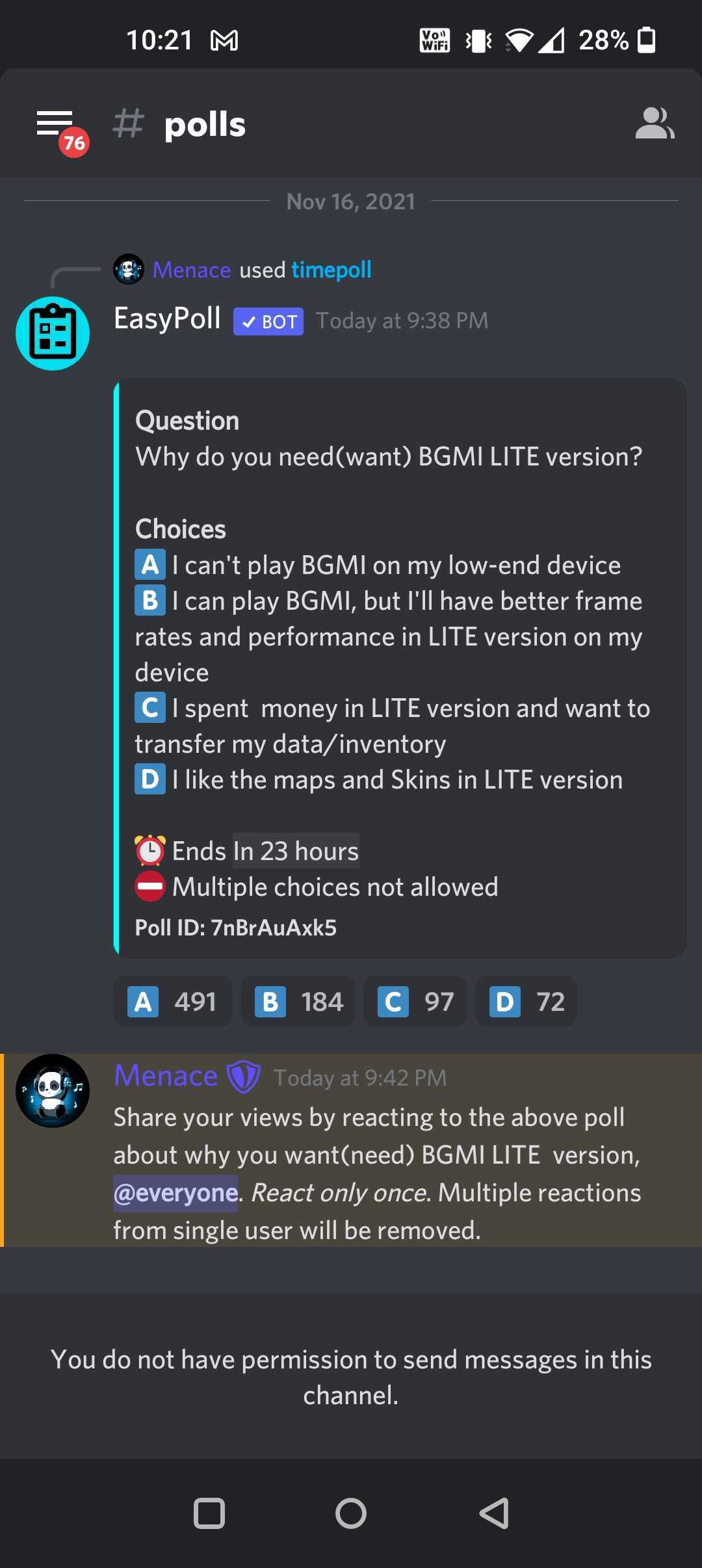In this image, we are presented with a screenshot taken from an Android mobile device. The status bar at the top of the screen displays various icons and indicators. On the left side, the current time reads 10:21. Moving to the right, we observe the following icons in sequence: VoWiFi (Voice over WiFi), vibrate mode, WiFi connectivity, network signal strength, and battery level.

Beneath the status bar, text appears in a question-and-answer format, asking: "Why do you need or want a BGMI Lite version?" Two response options are provided:
1. "I can't play BGMI on my low-end device."
2. "I can play BGMI, but I'll have better frame rates and performance in the Lite version on my device."

This screenshot appears to be taken from a settings menu or survey section within an application, aimed at gathering user preferences regarding the BGMI Lite version. The text suggests consideration for those with lower-end devices or those seeking improved performance.